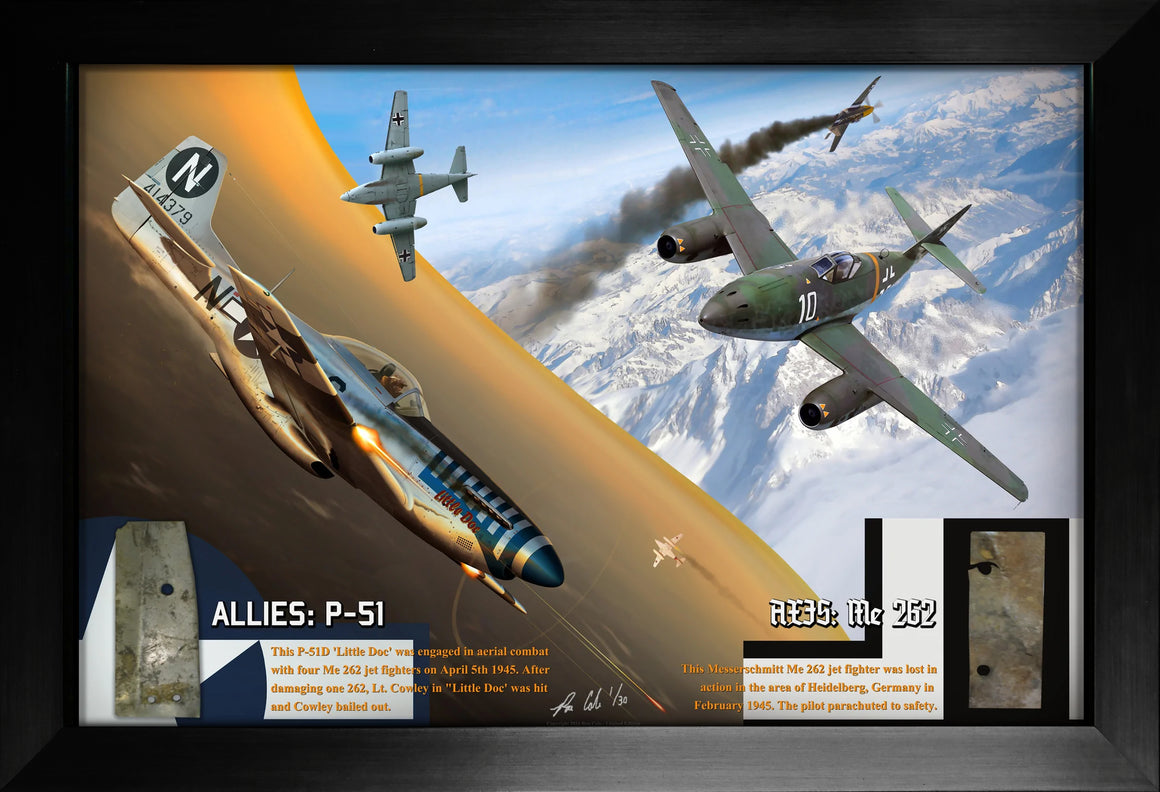The horizontal-rectangular, framed poster shows a detailed portrayal of World War II aircraft in an aerial scene. The dark gray frame encases an image taken from the sky, featuring a mix of bright blue sky and clouds, with snowy mountains visible below. The image foregrounds a brownish P-51 fighter plane, marked with the number 10 and what appears to be a missile on its side. This P-51, identified by the label "Allies P-51" in the bottom-left corner, seems to be flying level. Above it, another aircraft, an Me 262, marked with the number 414379 and labeled in the bottom-right corner, appears to be soaring over the P-51's right side. Two other planes can be observed in the background, adding depth to the dynamic aerial dogfight scene. The clarity of the image, with the bright and vivid lighting, enhances the realism and drama of this WWII aerial combat depiction.